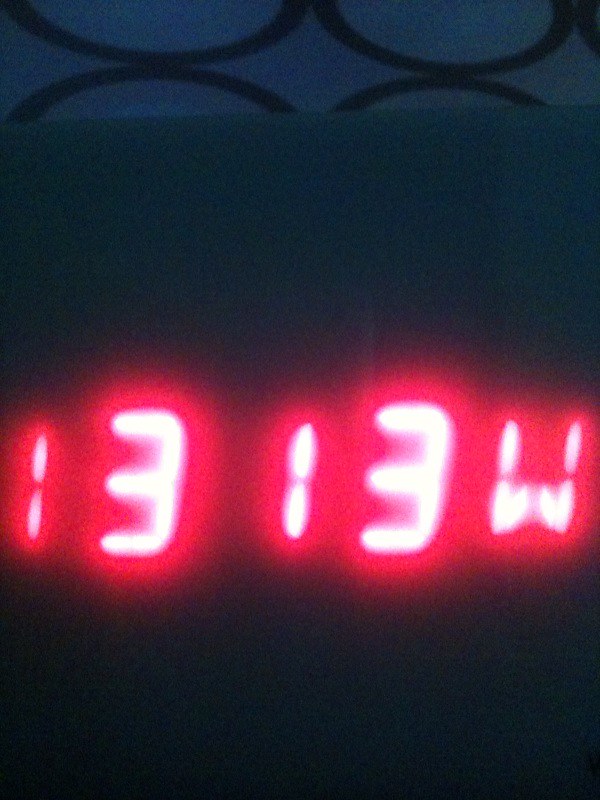The image is a close-up photograph in portrait mode, featuring an unclear object with digital numbers and letters displayed prominently in the center. The blurry-yet-bright display shows the sequence "1313W," where the numbers are white and surrounded by a vivid red glow. The background is predominantly dark, possibly black or a very deep blue, contrasting sharply with the illuminated figures. The threes appear slightly larger than the ones, adding to the distinctness of the display. At the very top of the image, there are faint half-circle designs that might be part of a fabric or furniture pattern, adding a decorative element to the scene.